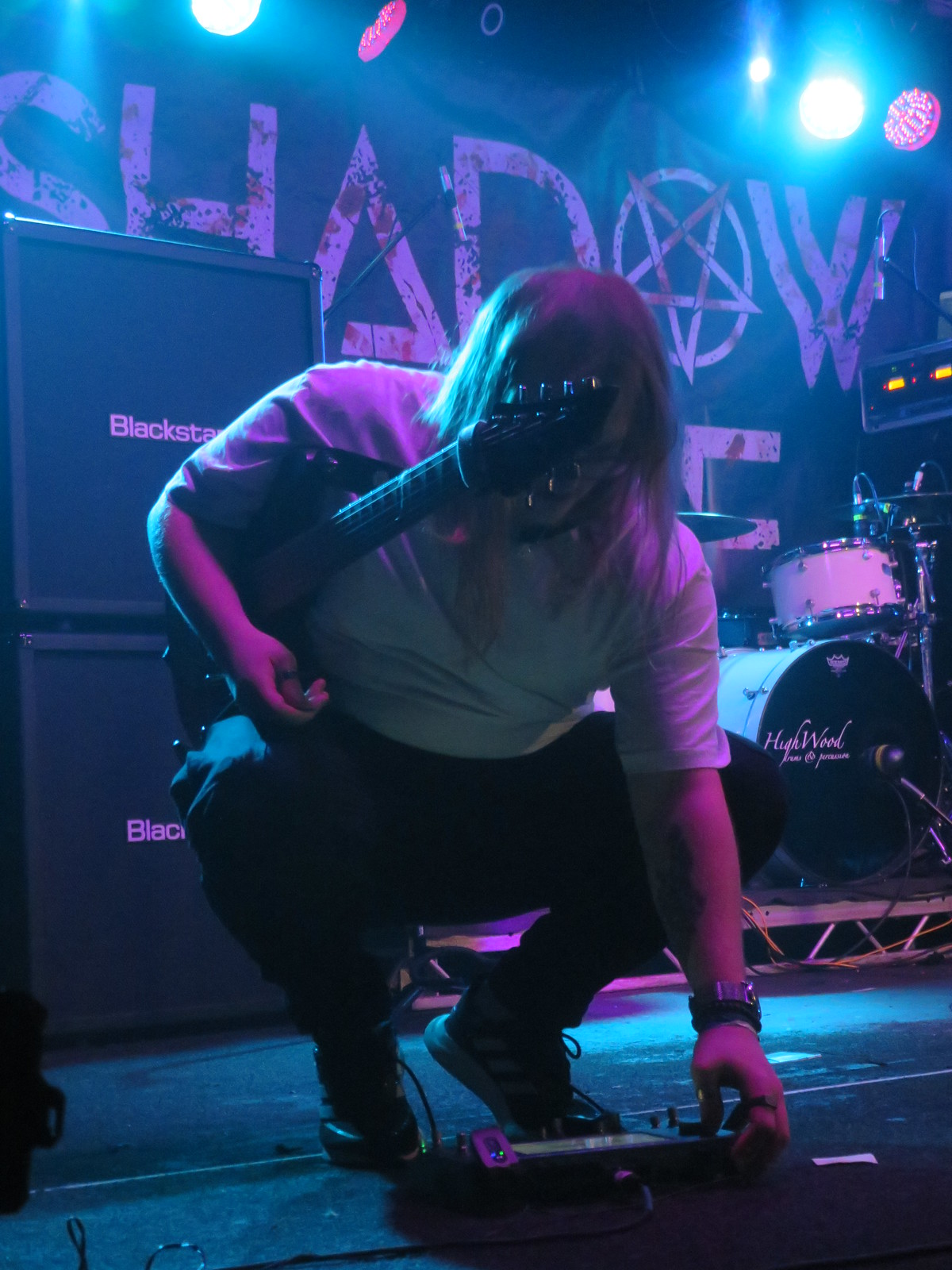In the image, a guitarist is kneeling on stage, adjusting electronic equipment at the bottom of the frame. The person, possibly a man but not clearly identifiable, has long, straight, light-colored hair falling over their face as they focus on the equipment. They're wearing a short-sleeved white t-shirt, black pants, and black and white high-top tennis shoes. The guitar is cradled under their right arm, partially obscuring their face. They are of a heavier build and are wearing glasses.

The backdrop features two large black speakers to the left, with the word "Blackstar" partially visible in white print. To the right, a white drum set labeled "Highwood" can be seen. Additionally, there's a black banner with the word "Shadow" at the top; the 'O' in the word is styled as a pentagram, hinting at a heavy metal or hard rock band, with the text appearing to be splattered in blood. The stage is bathed in blue and purple lighting, creating a dark, atmospheric indoor setting. There are no other people, such as audience members or bandmates, visible in the image.